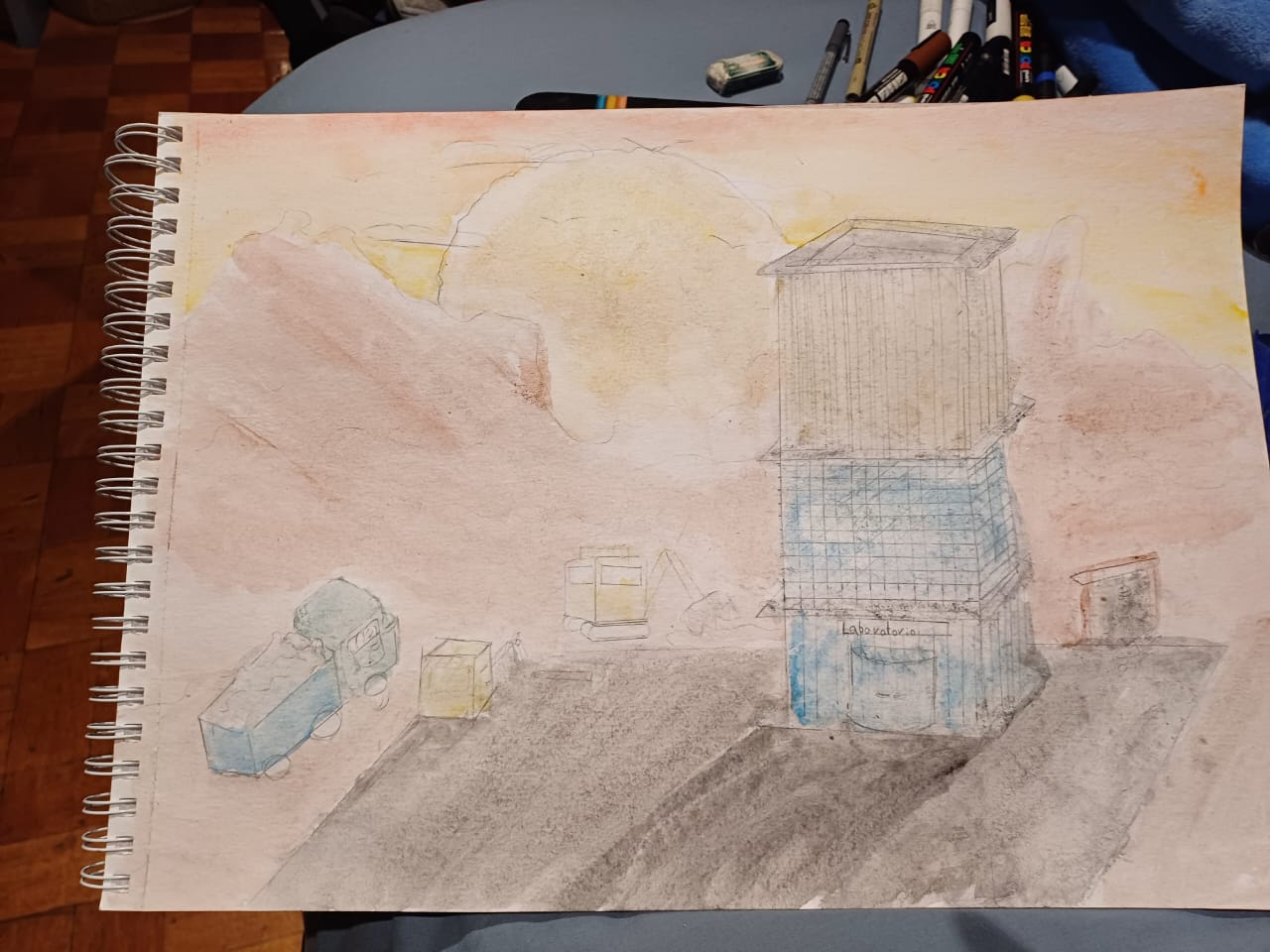The image appears to be a child's drawing depicting a three-story laboratory building labeled "Laboratory" at the top. The building has distinct slabs extending outward between each floor. Heavy equipment is featured prominently in the scene, including a truck with a large container on its back and at least one backhoe situated on a possibly concrete slab. The setting is a desert-like area on the outskirts, with a mountainous background and a setting sun. The depiction is housed in a spiral-bound notebook. In the foreground, there's a blue table with several markers on it, accompanied by a matching blue chair, all set against a parquet wooden floor.